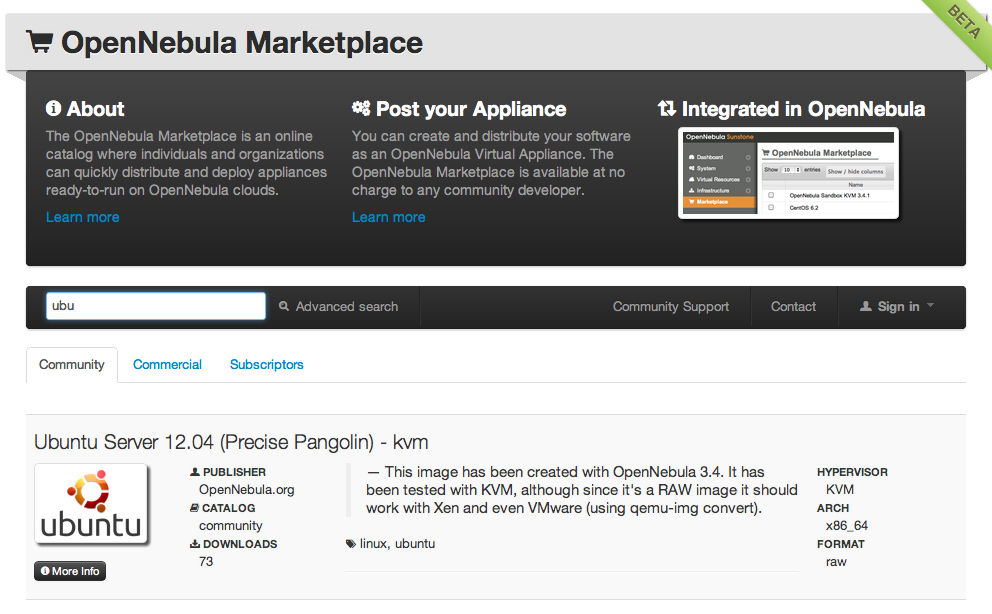The screenshot showcases the online interface of the Open Nebula Marketplace displayed on a desktop computer. The application screen features a sleek color scheme of dark gray, light gray, and white tones. At the top, a light gray horizontal bar spans the width of the screen. In the upper left corner of this bar, the text "Open Nebula Marketplace" is prominently displayed in black, accompanied by a shopping cart icon to its left. 

On the right side of this horizontal bar, a small green strip stands out with the word "Beta" inscribed. Below this, a darker horizontal frame is visible, containing white text and a white and gray rectangular section on its right side.

Further down, three distinct tabs are arranged horizontally, labeled "Community," "Commercial," and "Subscriptors," providing navigation options within the marketplace interface. The structured and clear layout facilitates smooth user interaction within the application.